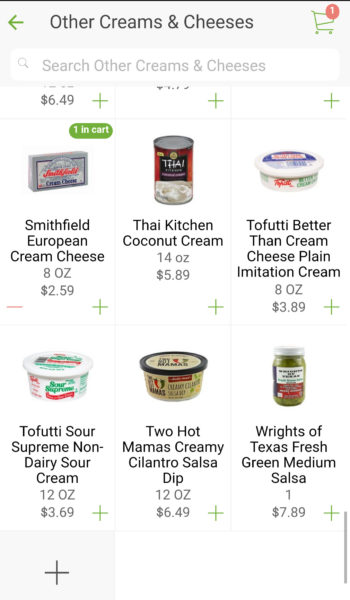This detailed caption provides a comprehensive overview of the web page's contents and layout:

---

This image showcases a web page promoting a sale on creams and cheeses. The top of the page is adorned with a gray header labeled "Other Creams and Cheeses." To the left, there is a green arrow pointing backward, and to the right, a shopping cart icon featuring an orange circle with the number "1" inside. Below the header, a search bar reads "Search Other Creams and Cheeses," which displays products when used.

Visible on the page are some product listings, though the top portions are truncated, showing only the price "$6.49" and green plus signs for adding items to the cart. Three key products are prominently displayed at the top:

1. **Smithfield European Cream Cheese** - 8 ounces priced at $2.59, with options to add or remove from the cart, highlighted by an orange minus sign.
2. **By Kitchen Coconut Cream** - 14 ounces canned, priced at $5.89, featuring an add option.
3. **Tofutti Better Than Cream Cheese, Plain Imitation Cream** - 8 ounces priced at $3.89 with an add option.

Additional products listed include:

- **Tofutti Sour Supreme Non-Dairy Sour Cream** - 12 ounces priced at $3.69.
- **Two Hot Mama's Creamy Cilantro Salsa Dip** - 12 ounces priced at $6.49.
- **Right to Texas Fresh Green Medium Salsa** - priced at $7.89.

At the very bottom of the page, there is a gray box with a central plus sign, likely indicating an option to load more products or add additional selections.

---